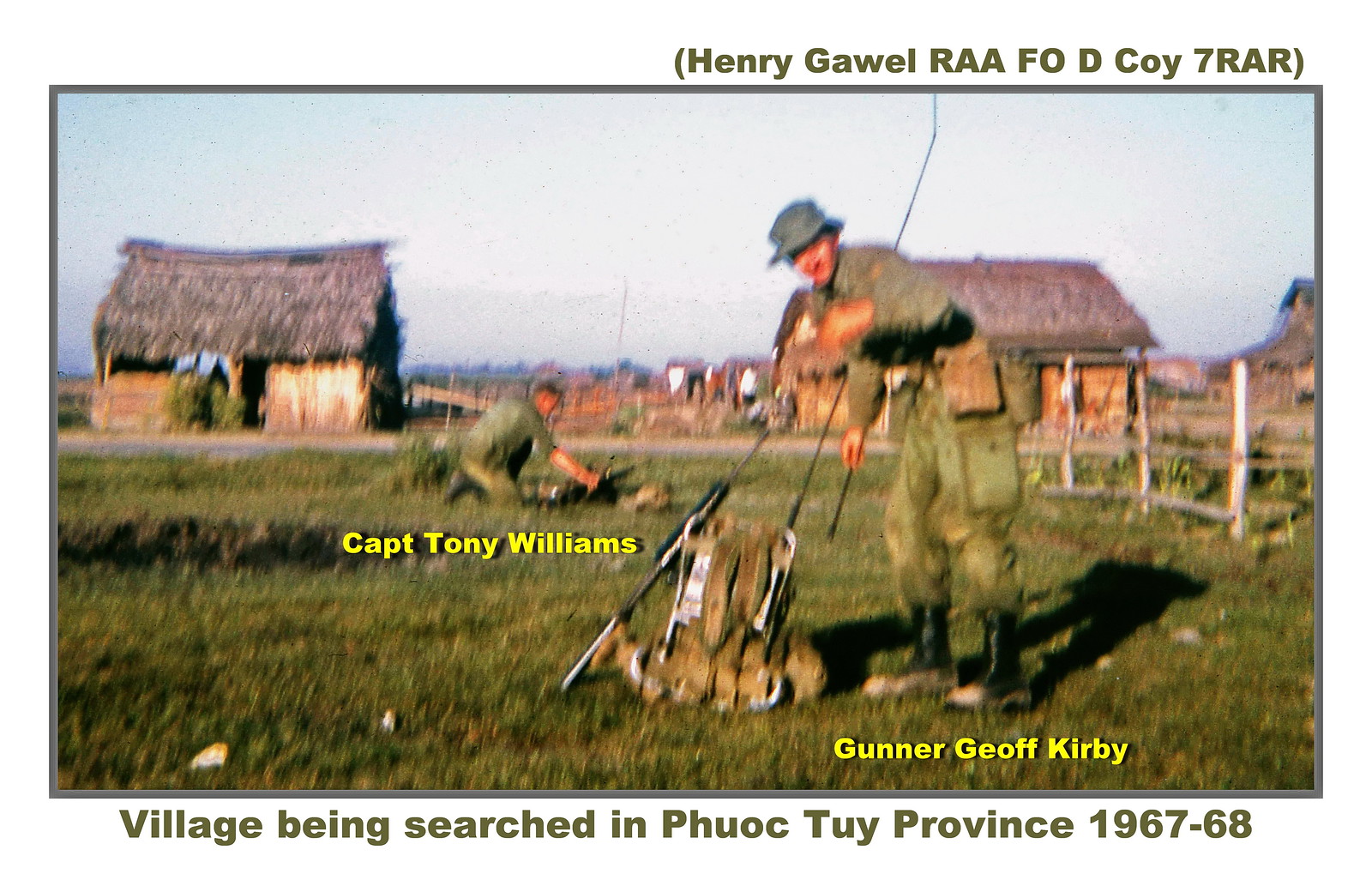A blurry historic photograph from the Vietnam War period, depicting a scene in Phuoc Tuy province between 1967 and 1968. The image shows a rural village with straw-thatched huts in the background and barren land leading to a grassy foreground. A small garden fence is visible on the right side. To the right of the center stands Gunner Jeff Kirby, who is facing the camera and dressed in a uniform, hat, and black boots with a pack on his left hip. He appears to be leaning over an indistinguishable object on the ground. Further in the background, to the left, Captain Tony Williams is kneeling, also in uniform and boots, similarly tending to an unidentifiable item. Captions in yellow letters under the figures identify them and a black-lettered title at the bottom reads, "village being searched in Phuoc Tuy province 1967-1968." Above the photo, in black letters, is inscribed "Hanuikawa RA AFOD KOI 7RAR." The sky is light blue, adding to the distinct Southeast Asian atmosphere.